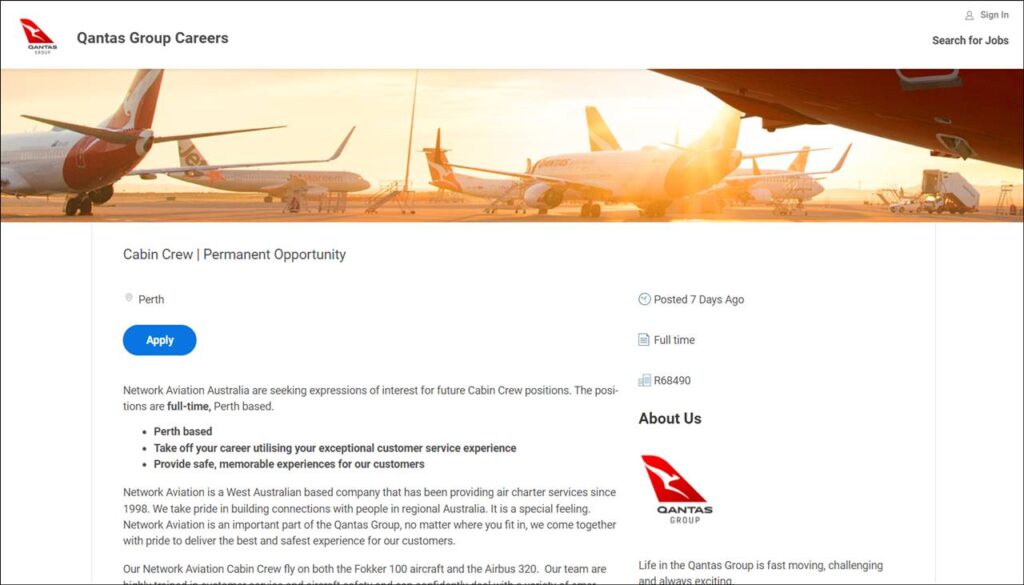Here’s a more detailed and cleaned-up descriptive caption for the image:

---

The screenshot captures the careers page of the Qantas Group website. In the top left corner, a small red icon is juxtaposed with the text "Qantas Group Careers" written in black. On the top right, there is a "Search for Jobs" option. Below this section, the central image features a fleet of airplanes stationed in what appears to be an aircraft parking lot during twilight hours, as the sky glows with a warm orange hue, indicating either sunrise or sunset. Beneath the photograph, the text announces "Cabin Crew Permanent Opportunity" with "Perth" mentioned in smaller text underneath. A prominent blue button labeled "Apply" urges potential candidates to take action. Below the button, there are three highlighted statements in dark or black text, each preceded by a dot: "Perth based," "Take off your career utilizing your exceptional customer service experience," and "Provide safe memorable experiences for our customers." To the right of these points, supplementary information indicates the job posting was uploaded seven days ago.

---